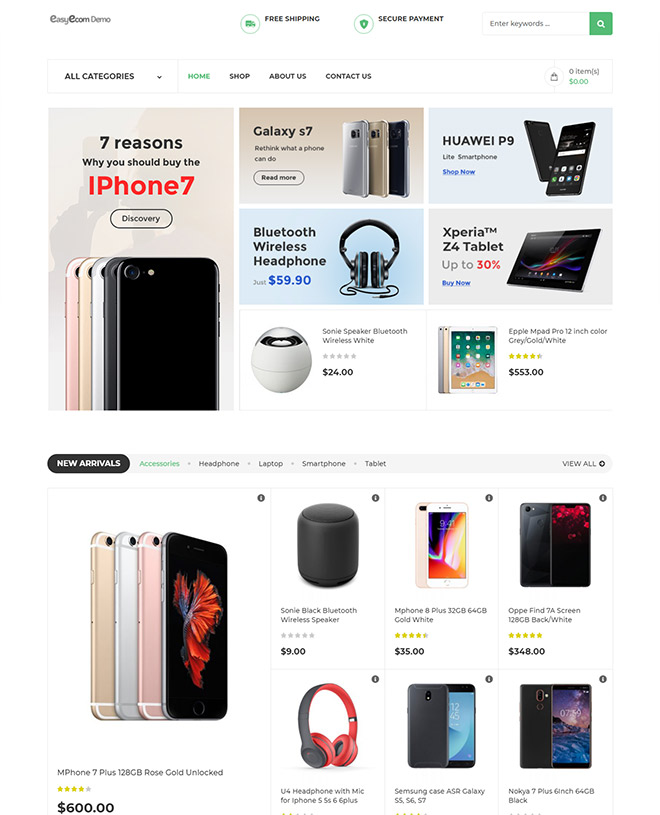This image depicts an e-commerce website specializing in the sale of smartphones, particularly iPhones. In the top left corner, the site's name is partially visible, ending with "demo," though it is too small to be distinctly read. Adjacent to the name is an icon of a green truck, accompanied by the text "Free Shipping." Another icon featuring a shield indicates "Secure Payment."

A search bar labeled "Enter keywords" is prominently displayed, with a green search button featuring a magnifying glass icon. Below the search bar, there is a navigation menu with options: "All Categories," "Home," "Shop," "About Us," and "Contact Us," with "Home" currently highlighted. Underneath this menu are promotional images and texts. 

One section titled "Seven Reasons iPhone 7" showcases various iPhone models. To the right, there are smaller listings for other products including "Galaxy S7," "HUAWEI P9," "Bluetooth Wireless Headphone," and "Xperia Tablet," each accompanied by a brief description and price details. The Bluetooth wireless headphones are listed along with a price, and the Xperia Tablet is highlighted with a 30% discount sticker. 

Further down, two items are displayed with their respective prices: one resembles an egg priced at $24, and another, which appears to be a tablet, has an unreadable price. The "New Arrivals" section at the bottom features a variety of phones and accessories, including headphones and speakers, further displayed for potential buyers.